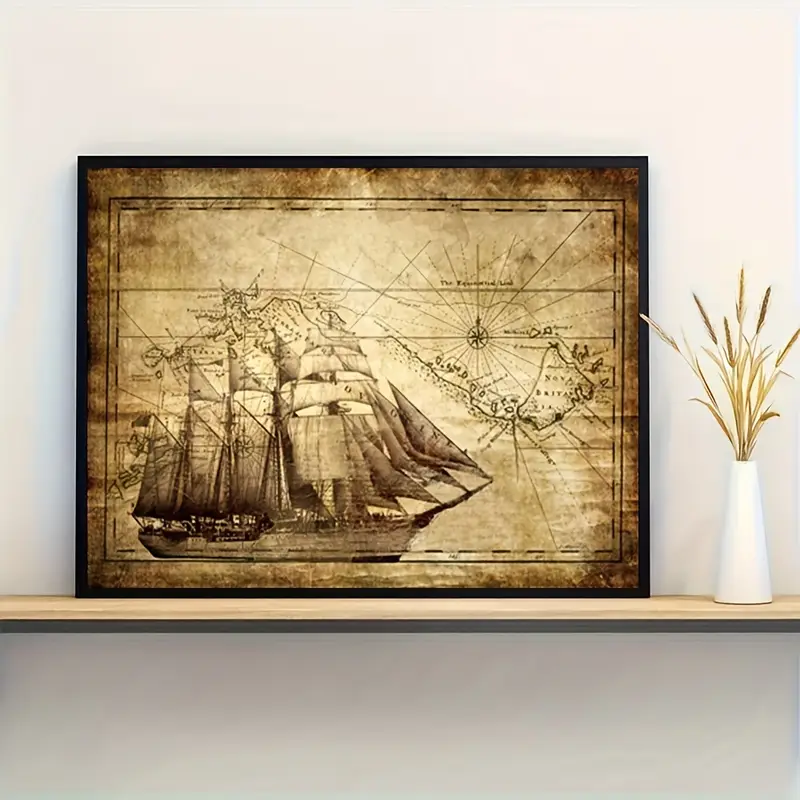This is an image of a framed painting resting on a long, wood-colored and gray sideboard against a white wall. The focal point of the painting is a large, multi-sailed ship from an era resembling the 1700s, possibly similar to vessels used by Christopher Columbus. The ship is surrounded by a nautical map featuring indistinct landmasses labeled with names like Nova Guinea and Nova Britain, and a prominent compass marks the background. The painting employs dark brown and beige tones for a realistic, sketched appearance. To the right of the painting on the sideboard, there is a small white vase with pale, grassy plants, potentially wheat or hay, adding a decorative touch to the scene. Overall, this image evokes the feel of a home’s living room mantle or sideboard adorned with maritime-themed decor.